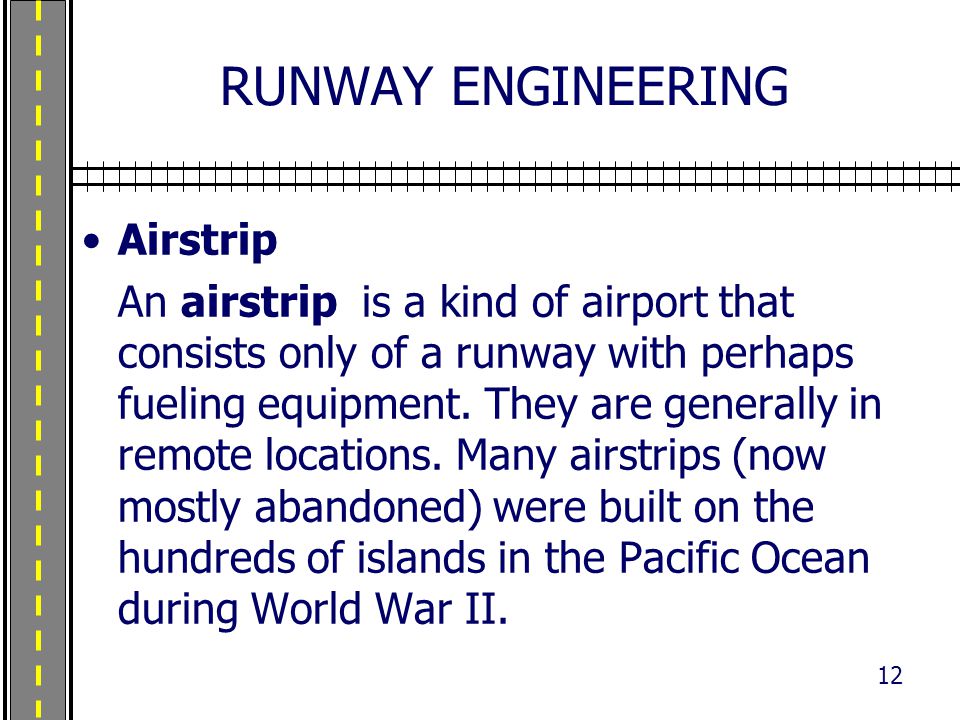The image resembles a PowerPoint presentation slide and features a vertically-oriented banner on the left depicting a road with yellow dashed lines and black bars at either end, occupying roughly an eighth of the screen. This banner is presumably representing an airstrip. At the top, the title reads "RUNWAY ENGINEERING" in large, uppercase, dark navy blue text. Below this title, there are simulated train tracks that run horizontally, acting as a divider. Further down, there’s a bullet point labeled "Airstrip," also in bold dark blue text. The caption following the bullet point explains: "An airstrip is a kind of airport that consists only of a runway with perhaps fueling equipment. They are generally in remote locations. Many airstrips, now mostly abandoned, were built on the hundreds of islands in the Pacific Ocean during World War II." The slide is minimal in color, predominantly featuring shades of gray with dark navy blue text, and the slide number "12" is positioned in the bottom right corner.